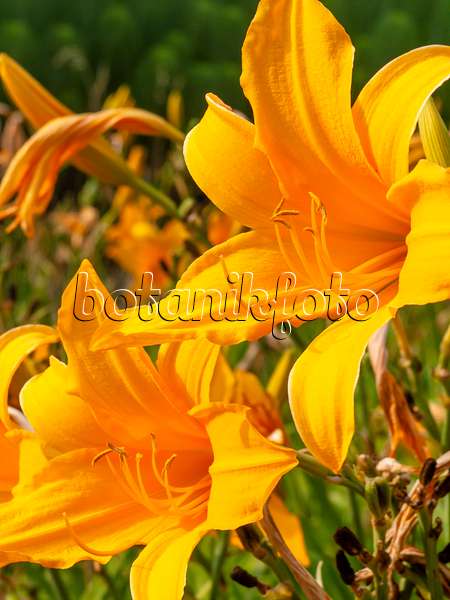This portrait-layout photograph features a close-up of two striking orange flowers with five or six petals each. The flowers are zoomed in, emphasizing the central shoots or pistils that extend prominently. Surrounding the main subject, a blurry background reveals a lush field of similar plants, portrayed with plentiful greenery and leaves, especially concentrated in a vivid green area at the top right. These secondary elements lend depth to the image. Centered within the frame is a cursive text overlay, "botanikfoto", in a color harmonizing with the flowers, serving as a watermark yet remaining legible. The overall effect is a vibrant and dynamic capture of colorful blossoms in a verdant field.